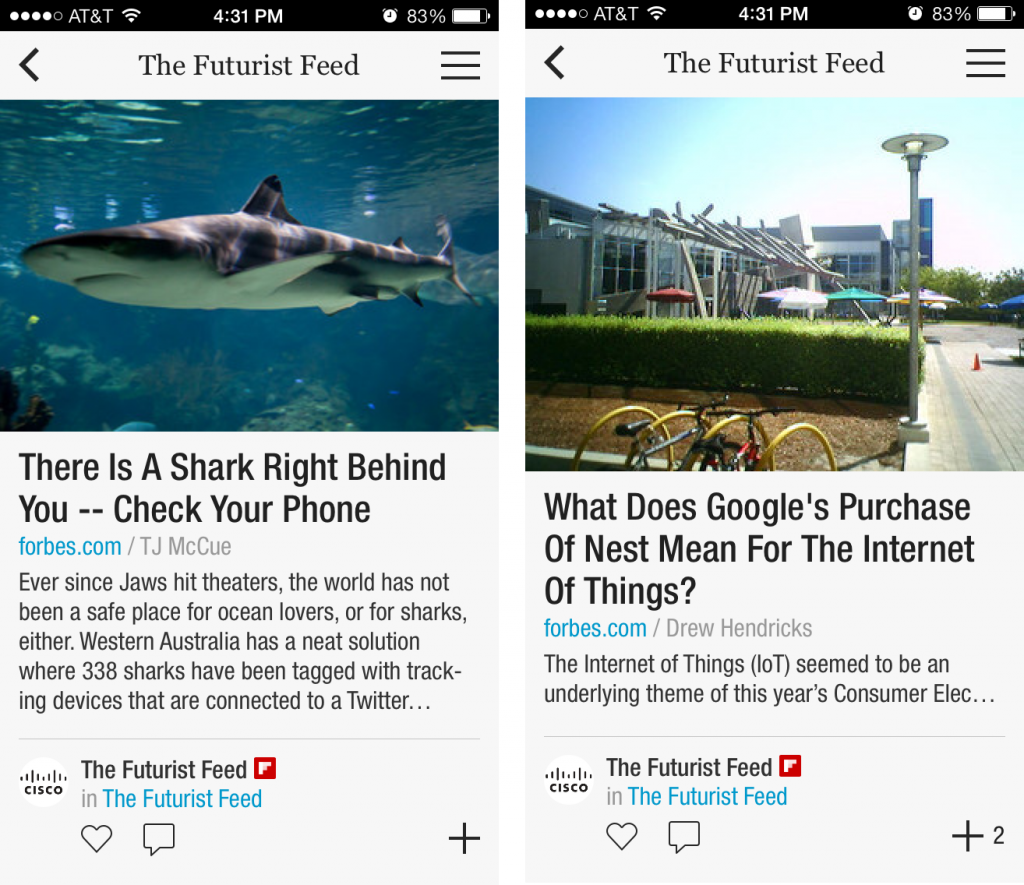Here is a detailed and cleaned-up caption for the given images:

---

The image showcases two screenshots from the Forbes.com section titled "The Futurist Feed," displayed on a cell phone. The first screenshot features an article adorned with a vivid underwater picture of a shark swimming amidst plants, accompanied by the bold headline: "There is a Shark Right Behind You. Check Your Phone." Authored by TJ McHugh, the article's subhead highlights the impact of the movie "Jaws" on ocean perceptions and describes a novel shark-tracking initiative in Western Australia, which connects 338 tagged sharks to Twitter updates. The display includes the Forbes logo, the Cisco logo, and interactive elements such as a like button, comment section, and sharing options.

The second screenshot presents another "The Futurist Feed" article, this time accompanied by an image showing bicycles in an urban setting with buildings and beach umbrellas in the background. The headline reads: "What Does Google's Purchase of Nest Mean for the Internet of Things?" Authored by Drew Hendricks, the article discusses the significance of the Internet of Things (IoT) at consumer electronics events. Similar to the first screenshot, it features the Forbes.com link, the Cisco logo, and engagement options including a heart for liking, a comment box, and an indicator showing that the article has been shared by two people.

Both articles offer insight into technological advancements and their societal impacts, underscored by the "The Futurist Feed" branding and the distinctive layout unique to Forbes.com.